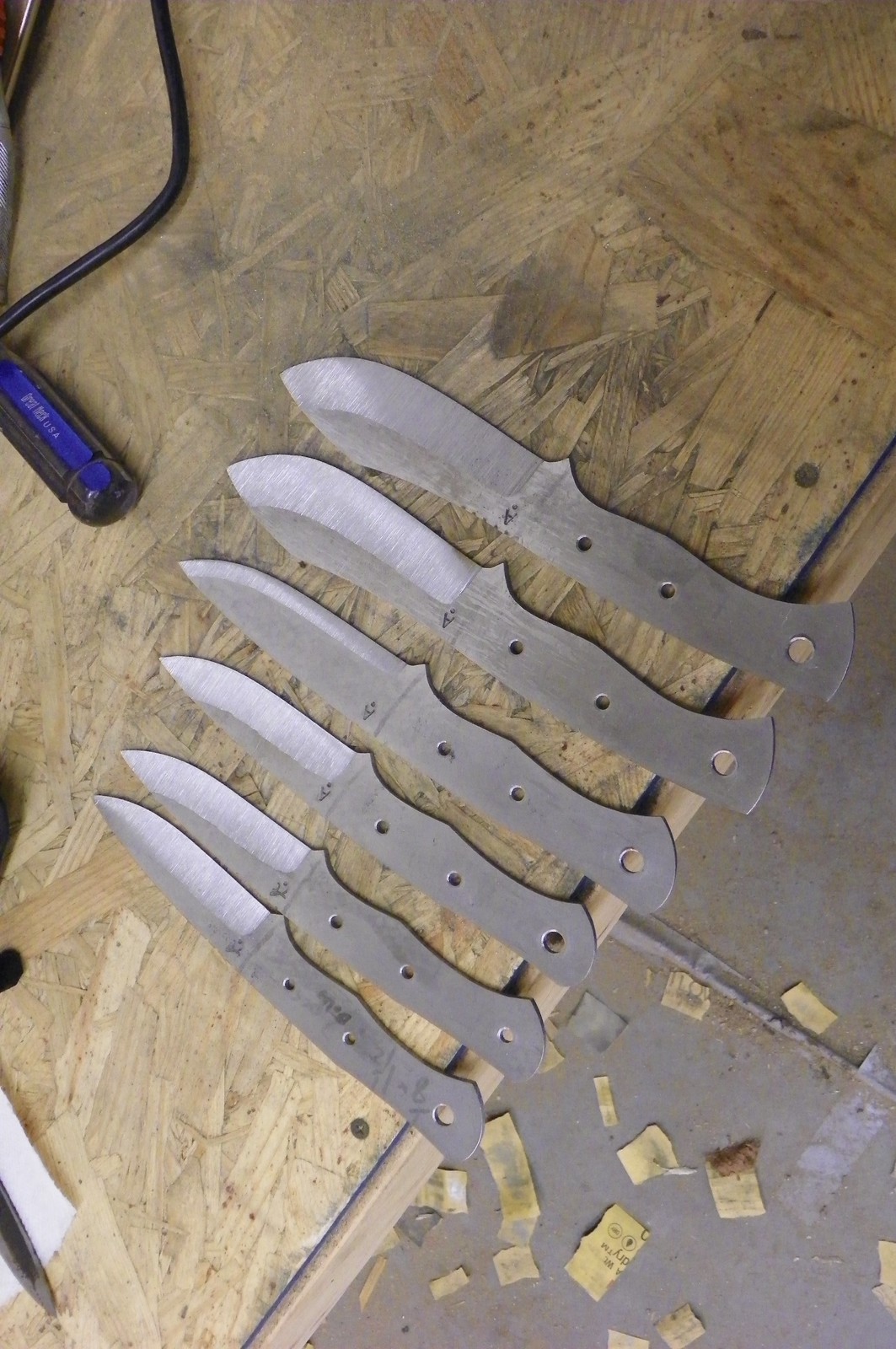This photograph captures an organized array of six unfinished knife blades in what appears to be a workshop setting. The vertically rectangular frame highlights the blades as the central focus, all neatly aligned on a piece of particle board. Each blade, silver in color, extends diagonally towards the upper left corner, creating a visually dynamic arrangement. The blades themselves vary in size and shape, with the first three being similar in dimensions, resembling steak knives, while the last three progressively increase in size, with shapes evocative of small swords or larger utility knives. The metallic shafts, awaiting their handles, feature three uniform holes designed for handle attachment. Notably, a dark blue-handled tool, likely a screwdriver, peeks from the top left, while the tip of a black pen is visible at the bottom left, subtly framing the knives and adding to the ambiance of a busy, tool-filled workshop.